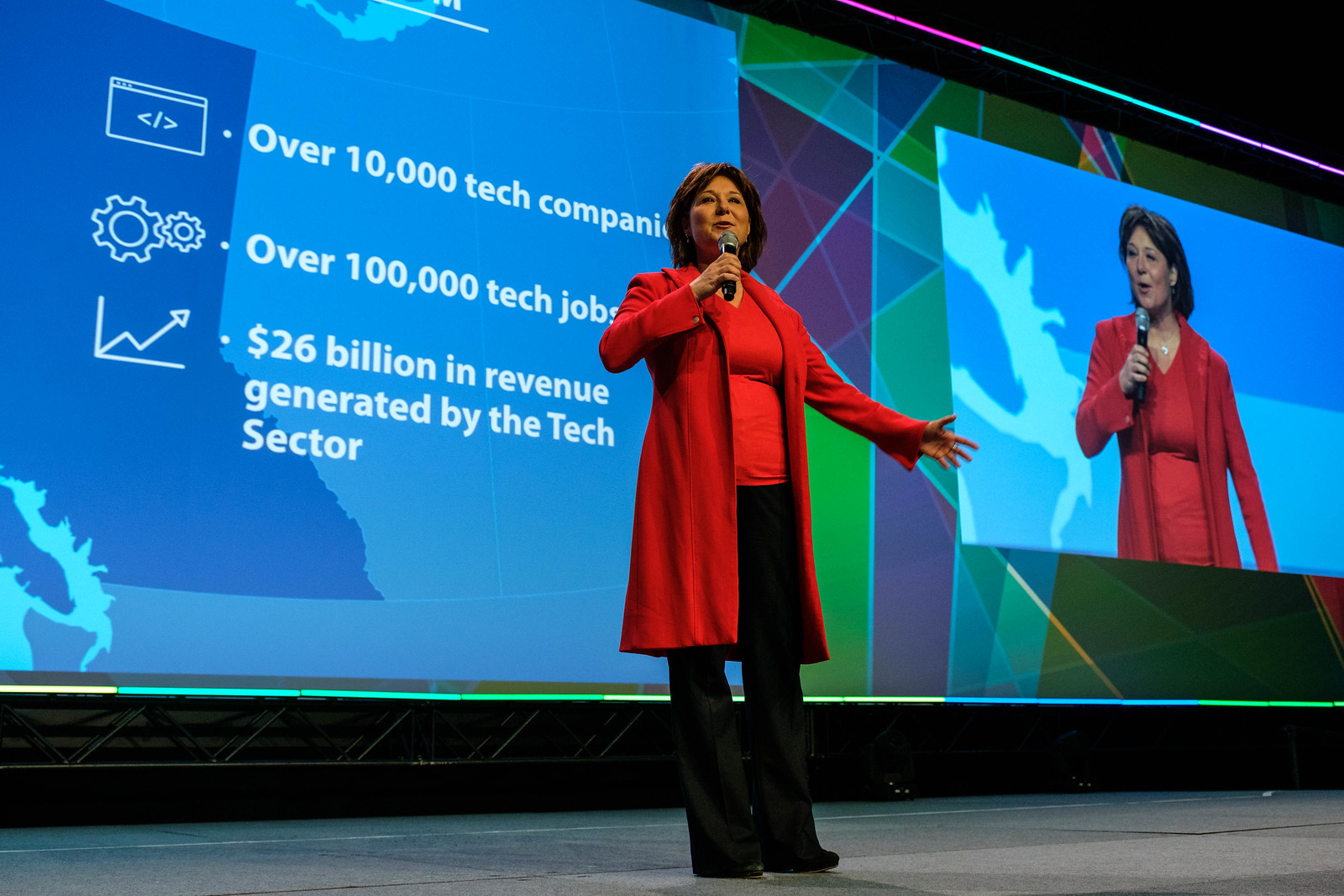In the center of the photo, a light-skinned woman with short hair stands on a hard, stone-like surface, likely on stage during an indoor presentation. She is dressed in a red top beneath a red jacket that extends just above her knees, paired with black pants and black shoes. In her right hand, she holds a portable microphone close to her face, and her left hand, adorned with a ring, is extended outward with fingers splayed. Behind her, occupying the left half of the image, is a PowerPoint presentation displayed on a screen. The presentation includes the following text: "Over 10,000 tech companies. Over 100,000 tech jobs. $26 billion in revenue generated by the tech sector." In addition, her image is also projected onto another screen on the right side of the photo. The colors in the background include various shades of blue, gray, black, red, green, pink, purple, and teal, contributing to the visual context of the presentation setting.